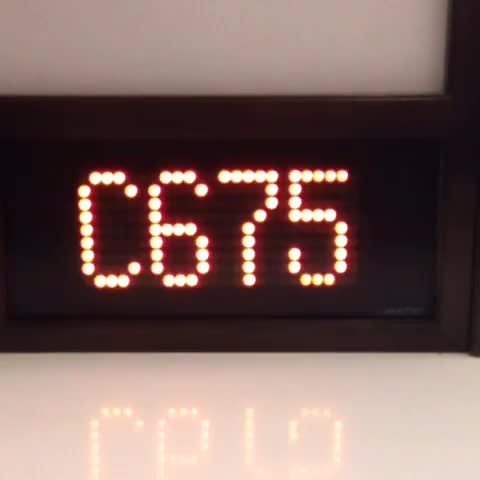In this image, we observe a digital display illuminated against a black background. The screen features white circular dots forming the characters "C675." Below this display, we see a reflective, shiny white surface that mirrors the displayed characters, but inverted. Consequently, the reflection shows "C," an upside-down "6," an upside-down "7," and an upside-down "5." The nature of the shiny surface is ambiguous; it could be part of a table, a shelf, or an extension of the equipment housing the digital screen, though the image provides no further context to identify it precisely.